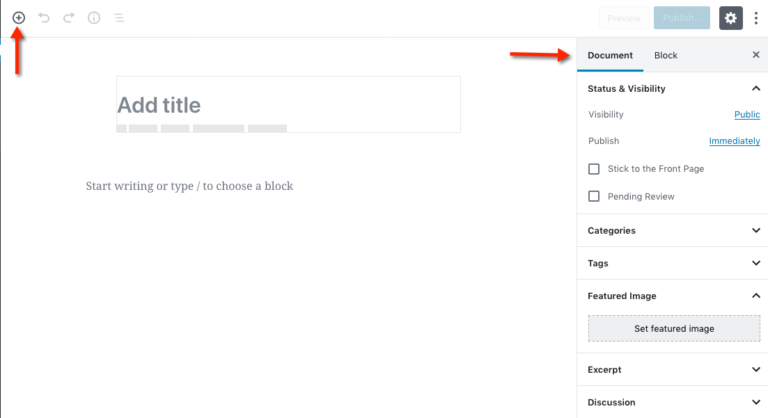Screenshot Description:

The screenshot depicts a white-background interface, presumably of a content management system. The key elements are spread between the right-hand and left-hand sides.

On the top-right corner, there is a white rectangle labeled "Preview" adjacent to a light blue rectangle labeled "Publish." Next to these buttons is a gray square containing a gear icon, followed by a vertically-stacked three-dot menu icon to the far right.

A light gray bar spans the screen beneath these top-right elements, featuring the words "Document" and "Block." "Document" is underlined in blue and has a red arrow pointing to it from the left. To the far right of this bar is an "X" icon.

Below this bar, it says "Status and Visibility" followed by sections labeled "Visibility" and "Publish." There is a small white checkbox beside the phrase "Stick to the Front Page," and another checkbox labeled "Pending Review" underneath.

Following these options are three rows titled "Categories," "Tags," and "Featured Image." The "Featured Image" section contains a rectangular box with a dotted border which says "Set Featured Image." Below these are two additional rows labeled "Excerpt" and "Discussion."

Over on the left side, in the top left-hand corner, there is a circled plus icon with a red arrow pointing up towards it. In the center of the screen, beneath this, there is placeholder text reading "Add Title," followed by the prompt "Start Writing or Type to Choose a Block."

The layout suggests a detail-oriented, user-centric interface designed for drafting and organizing content efficiently.